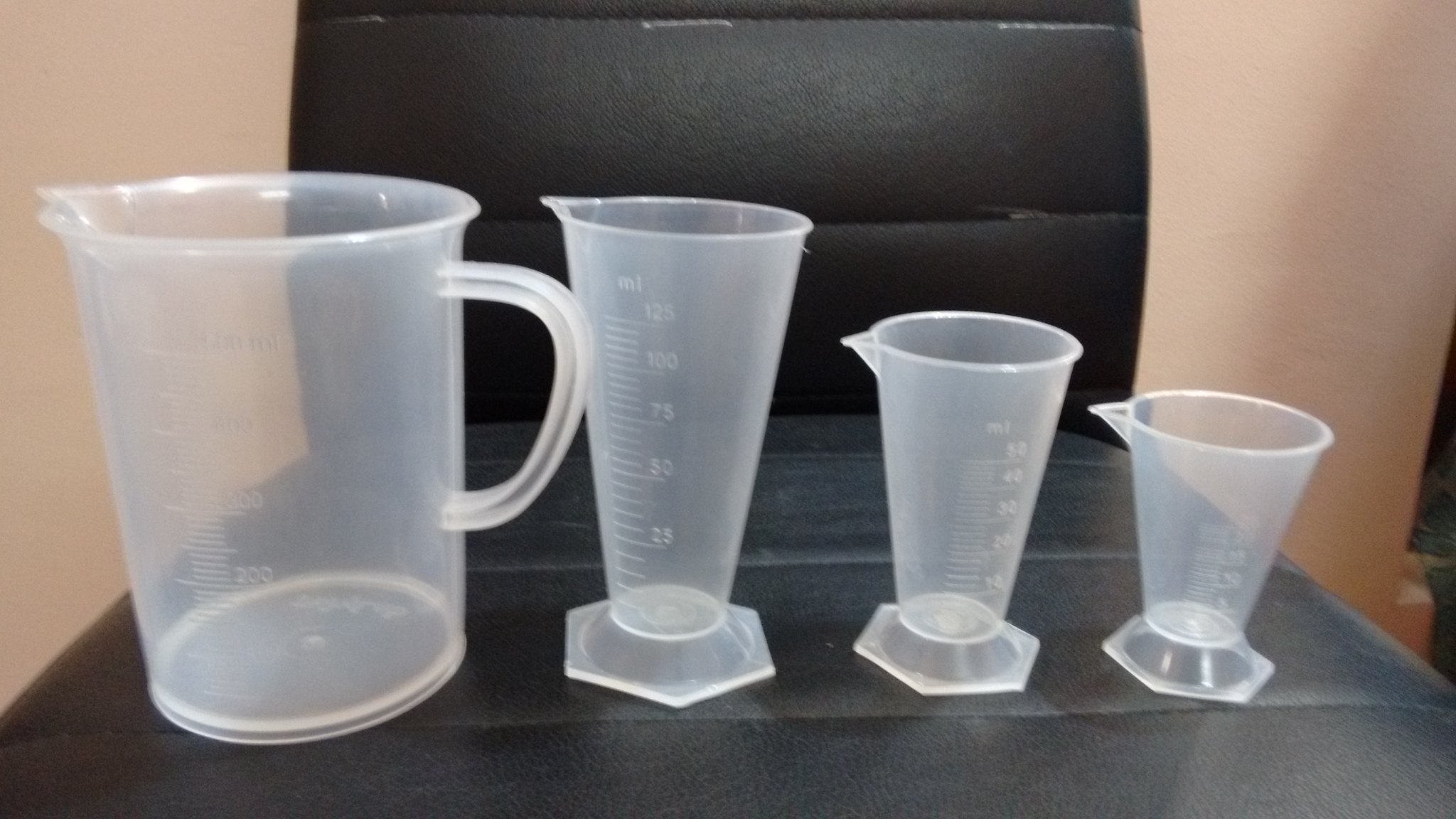The image depicts four clear plastic measuring devices resting on the seat of a black leather chair. The largest measuring cup, situated on the left, has a handle and is likely capable of holding between 600 to 800 milliliters. The second from the left is a cylindrical beaker with a six-sided base, holding approximately 125 milliliters, and features no handle but does have a pour spout. Next to it is a slightly smaller beaker, likely around 50 milliliters in capacity, similar in shape to its larger counterpart. The smallest vessel on the far right is also cylindrical and narrow, holding around 40 milliliters, but the exact volume is difficult to determine. All four measuring cups are intended for liquid measurement, with only the largest one differing in that it resembles a traditional pitcher with a handle for easy pouring.